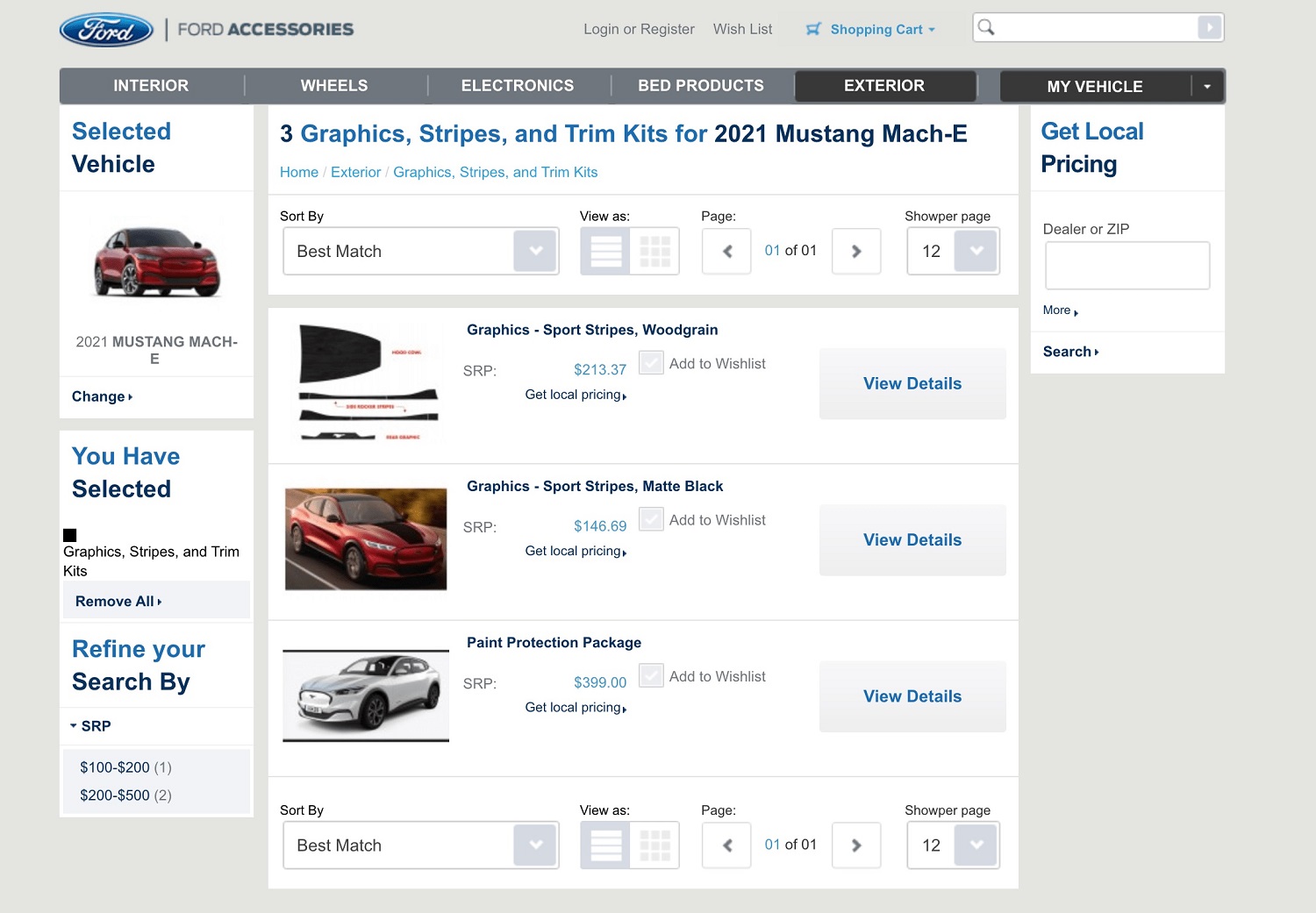The image depicts a web page from the Ford website. The top section features the Ford logo with "F-O-R-D-N-Y" emblazoned, set against a blue background. On the right side of the header, there are options labeled "Ford Accessories," alongside "Login or Register," "Wishlist," "Shopping Cart," and a search box.

Beneath this, there is a navigation bar with tabs for various categories such as Interior, Wheels, Electronics, Bed, Product, Exterior, and My Vehicle. The main content of the page highlights "3 Graphic Stripes and Trim Kits for 2021 Mustang Mach-E," with the text in blue and dark blue.

Below this headline, products are sorted by "Best Match," showcasing three items: 
1. "Graphic Sport Stripes Wood Grain" priced at $18.37, with additional details in blue text.
2. "Graphic Sport Stripes Matte Black" priced at $146.69.
3. "Paint Protection Package" priced at $399.

On the left side of the page, there is a section labeled "Selected Vehicle," featuring an image of a red Mustang Mach-E. Below this, a message states "you have selected Graphic Stripes and Trim Kits," with an option to remove all selected items.

At the bottom left corner, there's a "Refine Your Search" section with price ranges from $100 to $200 and $200 to $500. On the right side under the "My Vehicle" tab, there is an option to "Get Local Pricing" by entering a dealer or ZIP code.